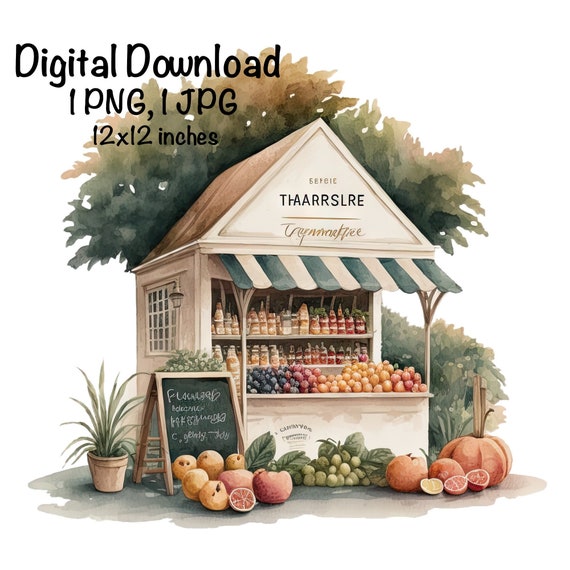This digital painting showcases a charming and meticulously maintained fruit farm stand, rendered in a watercolor-like style. The stand, predominantly white with a tan, smooth texture, features a sloped brown roof and a green and white awning that adds to its quaint appeal. Despite its modern and clean appearance, the exact materials of the stand — whether wood or otherwise — are indeterminate.

Above the stand, the image advertises its availability as a digital download in PNG and JPEG formats, sized at 12 by 12 inches. The text in the upper left corner reads: "digital download, 1 png, 1 jpg, 12 x 12 inches." The front of the stand is adorned with an array of small fruits, while larger fruits such as melons and pumpkins are stacked neatly in front, providing a vibrant and inviting display. The stand also contains various packaged products, possibly sauces, jams, or honeys, adding to the assortment.

A black chalkboard folding sign positioned at the front lists available items, written in an unfamiliar language. A tree in the background enhances the tropical, rustic charm of the scene. This artwork beautifully captures the essence of a bustling, yet serene fruit farm stand, blending modern digital techniques with traditional market aesthetics.